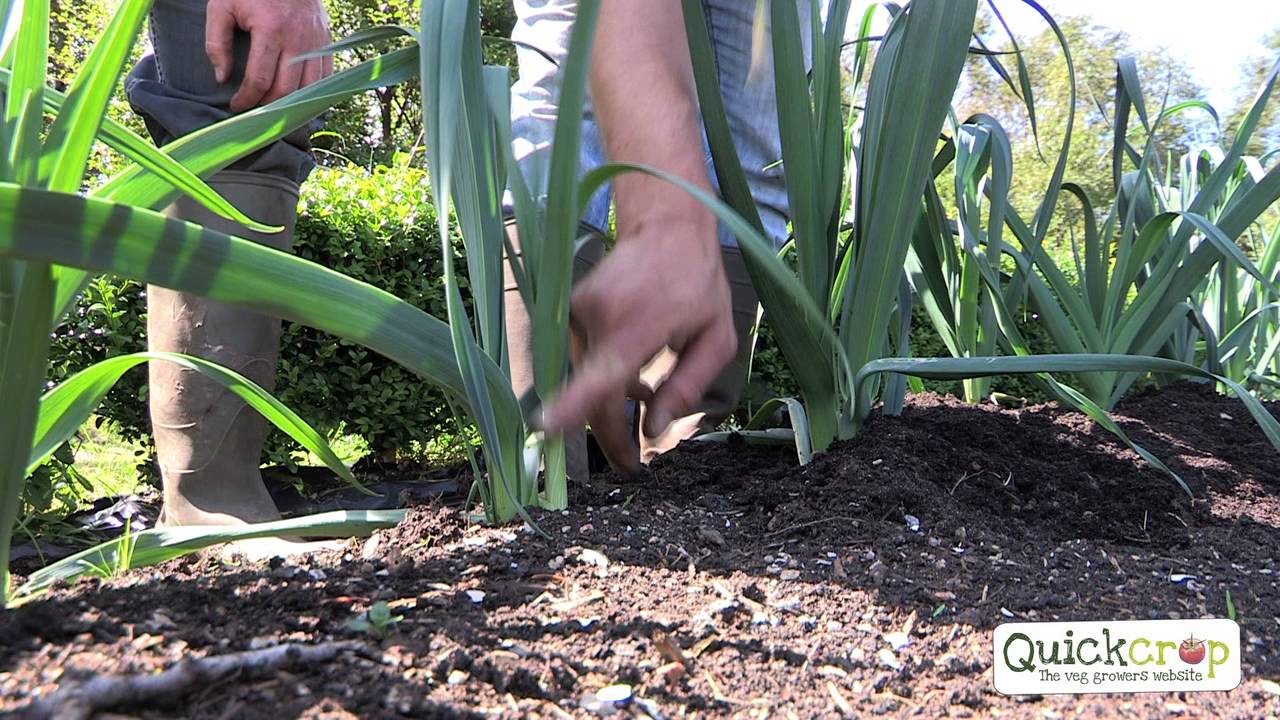This detailed photograph, presented in a rectangular landscape view, captures an up-close scene from a garden where crops, appearing to be leeks, are being grown in dark, moist soil. Central to the image are the legs and arms of two gardeners wearing Wellington boots and jeans; the individual on the left, wearing darker jeans, has his left hand resting on his knee, while the person on the right, donning lighter jeans, leans down to point at a crop with his right hand. The earthy foreground is dominated by thick green stalks emerging from rows of soil. In the background, beyond the figures, lies a hedge separating this garden section from additional greenery and trees, under a cloudy white sky. Prominently featured in the bottom right corner is a white rectangular box containing the text "Quick Crop" in varying shades of green, with the "O" in "Crop" depicted as an apple. Below, in smaller green text, reads "the veg growers website."